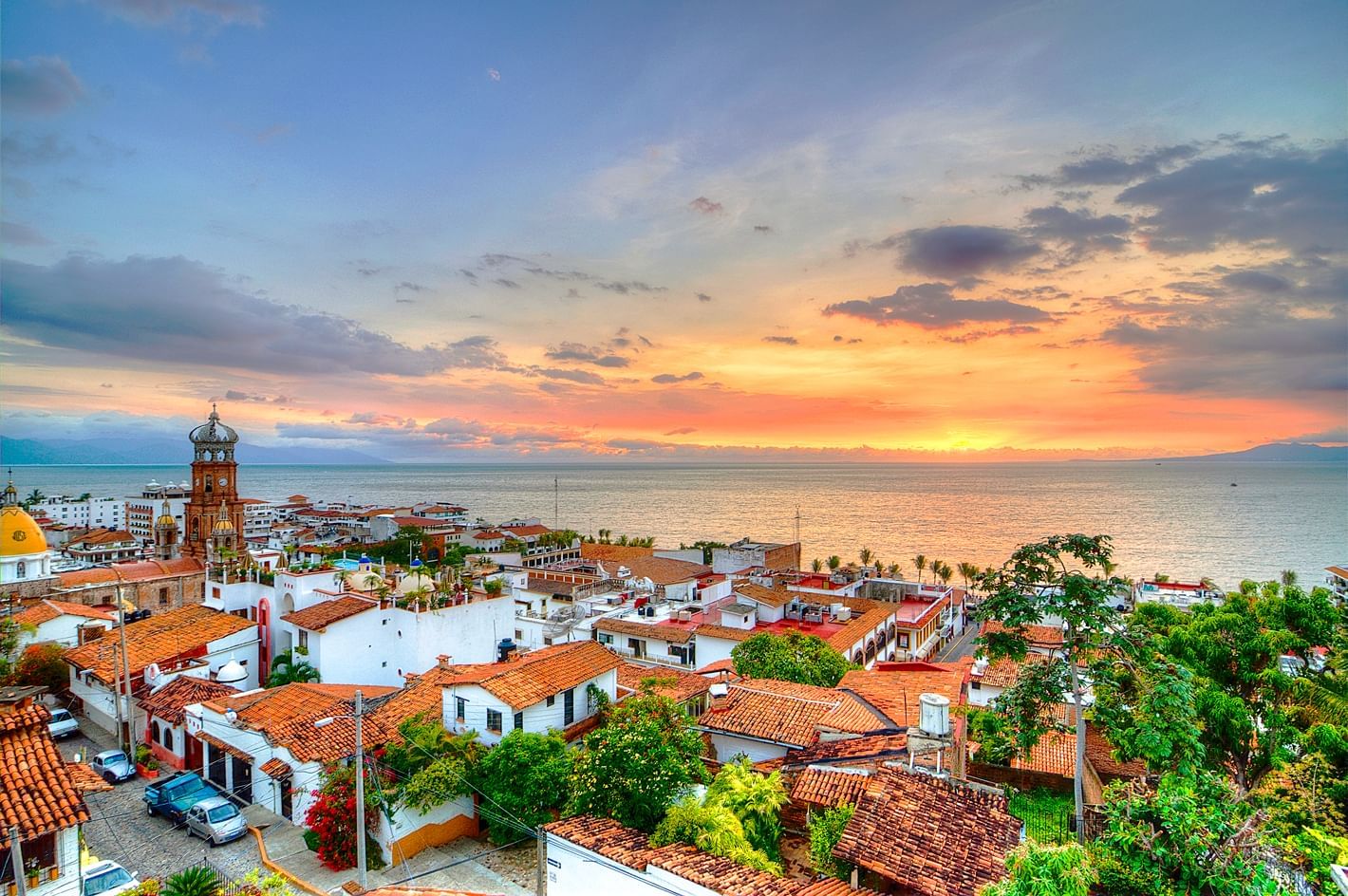The image captures a stunning sunset scene over a coastal town, showcasing an array of vibrant colors. The sky is a blend of deep blue fading into strips of pink, orange, yellow, and coral as the sun sets over the horizon. Streaks of pink and orange clouds add to the picturesque view. In the distance, the serene expanse of the ocean meets the horizon, creating a soothing backdrop.

The town is characterized by its white buildings with terracotta orange roofs, possibly a mix of homes and businesses, adding to the charm of the setting. Toward the left side of the image rises a small tower above the other buildings, serving as a noticeable landmark within the town. The bottom left corner reveals a glimpse of a city street where a few cars are parked, including noticeable white and blue cars.

Meanwhile, the bottom right corner features lush, green foliage, including leafy trees and what appears to be a rose bush, adding a touch of nature to the urban landscape. Additionally, the outline of a distant mountain is discernible on the very right, completing the harmonious blend of natural and architectural beauty in this sunset scene.